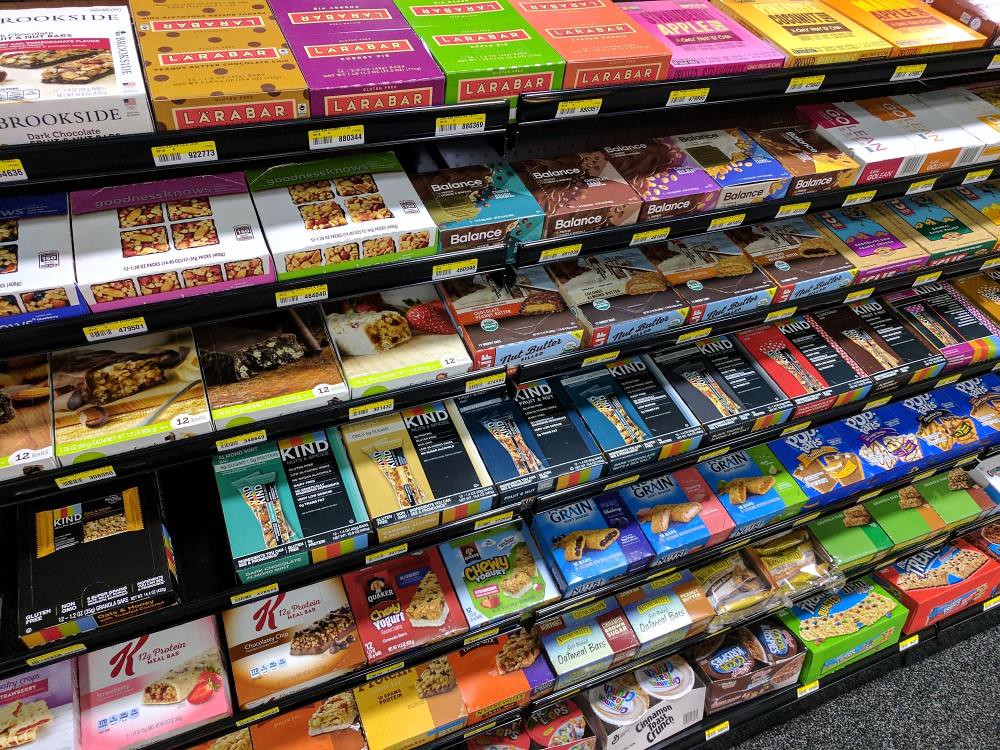The image captures a well-organized store shelf featuring a variety of products. On the top left corner, there is a box of Brookside Dark Chocolate with white packaging. To the immediate right of the Brookside box, there is an orange and dark brown package of Larabar, clearly labeled as "LARABAR." Next to it, another Larabar can be seen, this time in purple packaging. Each item on the shelf has a corresponding price tag positioned beneath it, facilitating an easy shopping experience for customers. The shelves are neatly arranged, highlighting the attention to presentation within the store.